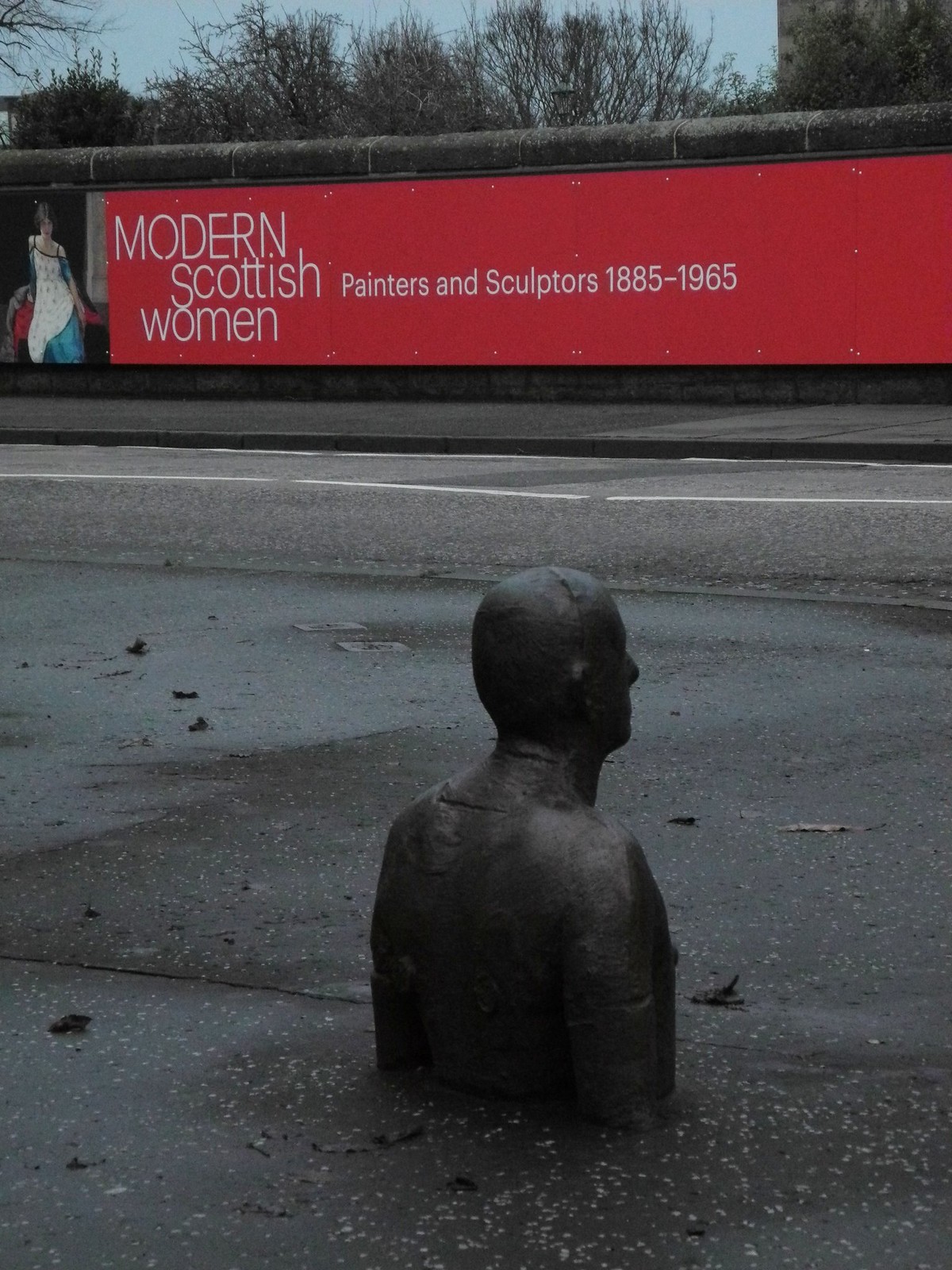The color photograph, in portrait orientation, showcases a surreal street view dominated by a remarkable bronze statue of a man. This statue is visible from the top of his head down to mid-chest, and it appears as though he is emerging—or submerged—from the asphalt pavement. The man's figure faces away from the viewer, toward the right side of the image, giving an impression of being sunken into or rising out of the road. Surrounding the statue is a gray asphalt street that stretches horizontally from the left to right edges of the photograph. Behind this, a dark gray short wall supports a red advertisement poster that spans the entire width. The poster features a color painting on its left side and white text to its right, which reads: "Modern Scottish Women, Painters and Sculptors, 1885-1965." The background of the image reveals a landscape of bare-branched trees under a clear blue sky. The scene blends photographic realism with special effects, portraying a unique and evocative piece of art.